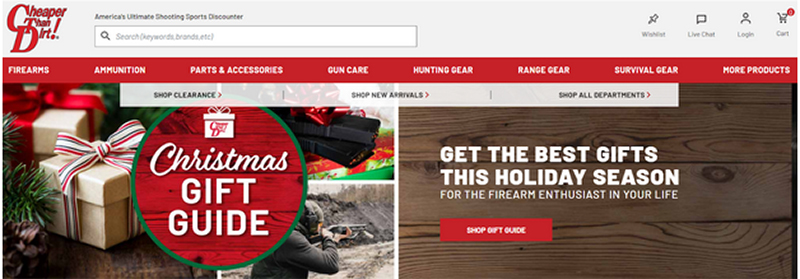This image depicts a horizontal strip from a website, prominently longer than it is tall, which appears to be an online store dedicated to shooting sports and related merchandise. In the top left corner, the store's logo "Cheaper Than Dirt!" is displayed in bold red text with an exclamation point. Below this, the tagline reads "America's Ultimate Shooting Sports Discounter." 

Beneath the tagline is a search bar prompting users to "search keywords, brands, etc." To the right of the search bar, four clickable options – Wish List, Live Chat, Login, and Cart – are neatly aligned. The Cart icon features a small red circle with the number zero, indicating no items in the cart.

Underneath, a horizontal navigation menu offers categories in white font against a contrasting background. The categories include Firearms, Ammunition, Parts & Accessories, Gun Care, Hunting Gear, Range Gear, Survival Gear, and a catch-all "More Products."

A secondary white band contains three clickable links: "Shop Clearance," "New Arrivals," and "Shop All Departments," each accompanied by a red arrow pointing right.

The focal point below the bands is an image on the left depicting festive packages underneath a Christmas tree, ammo cartridges adorned with ribbons, and an individual shooting. Overlaying this image is a circular badge labeled "Christmas Gift Guide."